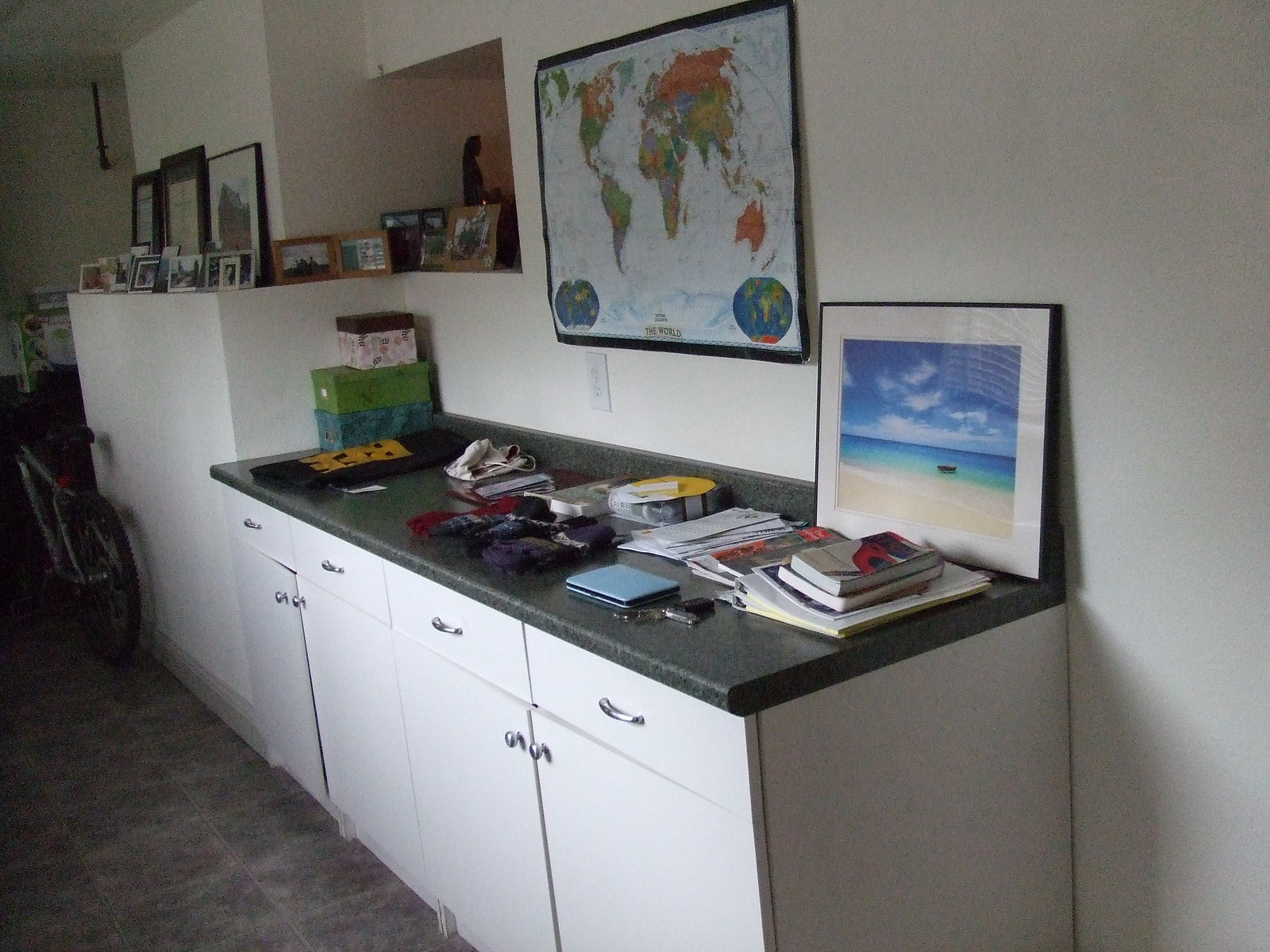The image depicts the interior of a spacious, enclosed room, resembling a converted garage. The walls are finished with white drywall, and the floor is covered in gray tiles. The back wall is lined with white cabinets featuring various storage options. The cabinet doors, adorned with circular silver knobs, open outward, while the white pull drawers have sleek, banded silver handles. Above the cabinets, a dark gray, speckled laminate countertop spans the length, cluttered with stacks of papers and a couple of books. In one corner, a green box, a turquoise box, and a smaller white-and-red-lid box are visible. Leaning against the countertop is a framed poster, depicting a serene beach scene with turquoise water, a blue sky, white clouds, and a boat. The poster has a black frame with a white inner border. Adjacent to it, mounted on the wall, is another poster showcasing a multicolored world map.